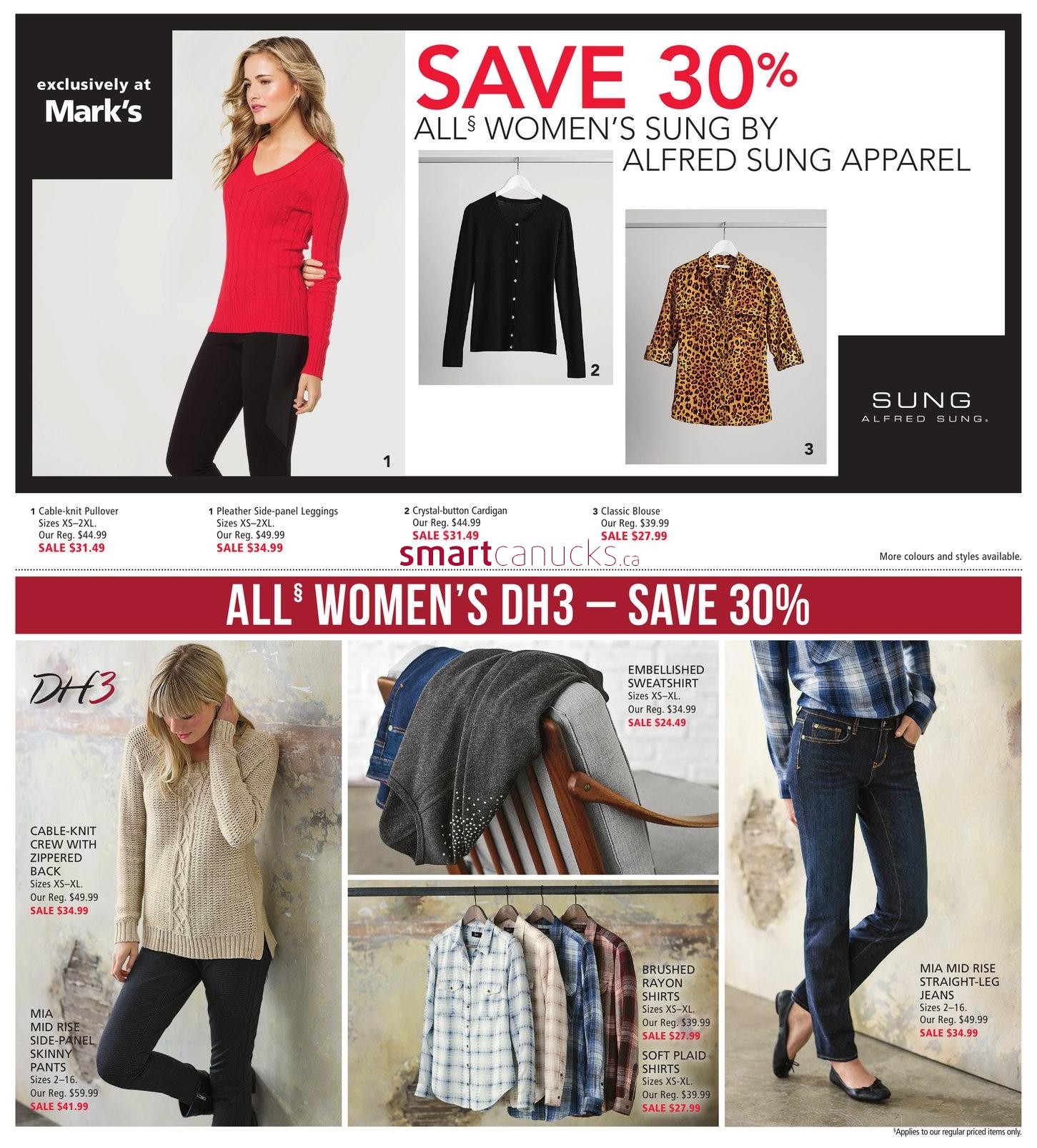**Detailed Promotional Caption:**

Discover incredible savings at Marks with their latest promotion on women's apparel by Alfred Sung and DH3. 

**Top Half Promotion:**

- **Main Banner:**  
  - A bold promotional banner announces a fantastic 30% discount on all women's apparel by Alfred Sung. The text "Save 30%" is prominently displayed in large, striking red font, with "All Women's Sung by Alfred Sung Apparel" written just below it.

- **Product Images:**
  - **Left Image:** 
    - A woman with long, wavy blonde hair models a bright red knit pullover sweater, paired with black leggings. She stands against a plain background, exuding casual elegance.
  - **Middle Image:** 
    - A black, long-sleeved cardigan with buttons, elegantly draped on a hanger against a white background, showcasing its classic design.
  - **Right Image:** 
    - A stylish leopard-print blouse with three-quarter sleeves is prominently displayed on a hanger, highlighting its trendy appeal.

**Bottom Half Promotion:**

- **Secondary Promotion:**
  - An additional 30% discount on all women's DH3 apparel is highlighted with the text "All Women's DH3 Save 30%" also displayed in eye-catching red font.

- **Product Images:**
  - **Top Left Image:** 
    - A woman with straight blonde hair models a beige crew neck knit sweatshirt featuring a zippered back. She leans effortlessly against a textured wall, paired with black pants for a chic look.
  - **Middle Image:** 
    - A gray embellished sweatshirt is draped over the back of a wooden chair, showcasing its detailed design and cozy appeal.
  - **Bottom Center Image:** 
    - A row of brushed flannel shirts in various plaid patterns is neatly displayed on a rack, perfect for a versatile and stylish wardrobe.
  - **Bottom Right Image:** 
    - An image of a woman wearing a blue and white plaid shirt paired with dark blue mid-rise jeans. She stands confidently with one hand in her pocket, highlighting the flattering fit of the Mia Mid-Rise Straight Leg Jeans.

**Product Listings and Prices:**

- Cable Knit Pullover Sweater: $31.49
- Pleather Panel Leggings: $34.99
- Crystal Button Cardigan: $31.49
- Classic Leopard Print Blouse: $27.99
- Crew Neck Knit Sweater with Zippered Back: $34.99
- Mia Mid-Rise Side Panel Skinny Jeans: $34.99
- Gray Embellished Sweatshirt: $24.49
- Brushed Flannel Shirts (various plaids): $24.49 each
- Mia Mid-Rise Straight Leg Jeans: $34.99

Experience these incredible savings on stylish and versatile women's apparel at Marks, and elevate your wardrobe with timeless pieces from Alfred Sung and DH3.